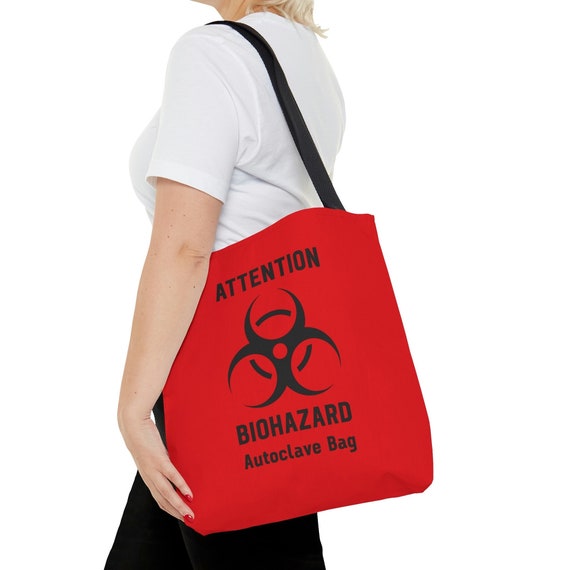This image is a striking advertisement featuring a woman in a minimalist, clean setting. The white background emphasizes the stark simplicity and focus of the composition. The model, seen from the side and roughly from the neck down to her thighs, has blonde hair and wears a white short-sleeved shirt paired with black pants. Her complexion is Caucasian, and she sports red fingernails that match the color theme of the focal object in the picture—a large red tote bag with a black strap, slung over her left shoulder.

The red bag prominently displays bold black text that reads: "Attention: Biohazard Autoclave Bag." Centered on the bag is the universally recognized biohazard symbol, a striking black emblem consisting of three intersecting circles forming a triangular shape. The model's left hand supports the bottom of the bag, emphasizing its significant presence. The overall design suggests that the bag is meant to be eye-catching, potentially used as a statement or conversation piece, perhaps even marketed playfully despite the serious connotations of its design. The stark white background further isolates and highlights the bag, making sure your attention is undivided.